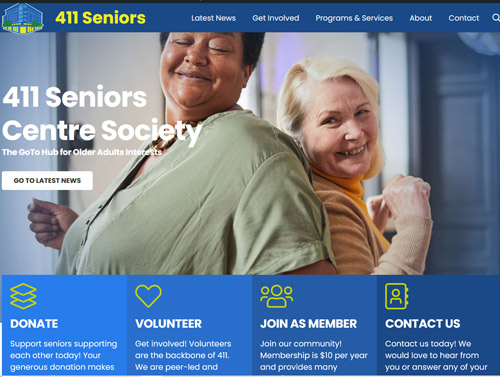The image prominently features the logo and name of the 411 Seniors Centre Society, positioned at the top left corner. The image lays out various navigation links and calls to action including the latest news, ways to get involved, programs and services, information about the organization, and contact details. 

In smaller text, the image describes the 411 Seniors Centre Society as the central hub for older adult interests. It encourages viewers to explore the latest news, make a donation, volunteer, or join as members. A strong emphasis is placed on the vital role of volunteers, stating that they are the backbone of the organization. 

The image also highlights that membership, which costs $10 annually, comes with numerous benefits. Finally, it invites potential members and volunteers to get in touch for more information or with any questions, promoting a community-oriented and supportive environment. 

The overall message underscores the importance of mutual support among seniors and the value of community involvement through volunteering and donations.